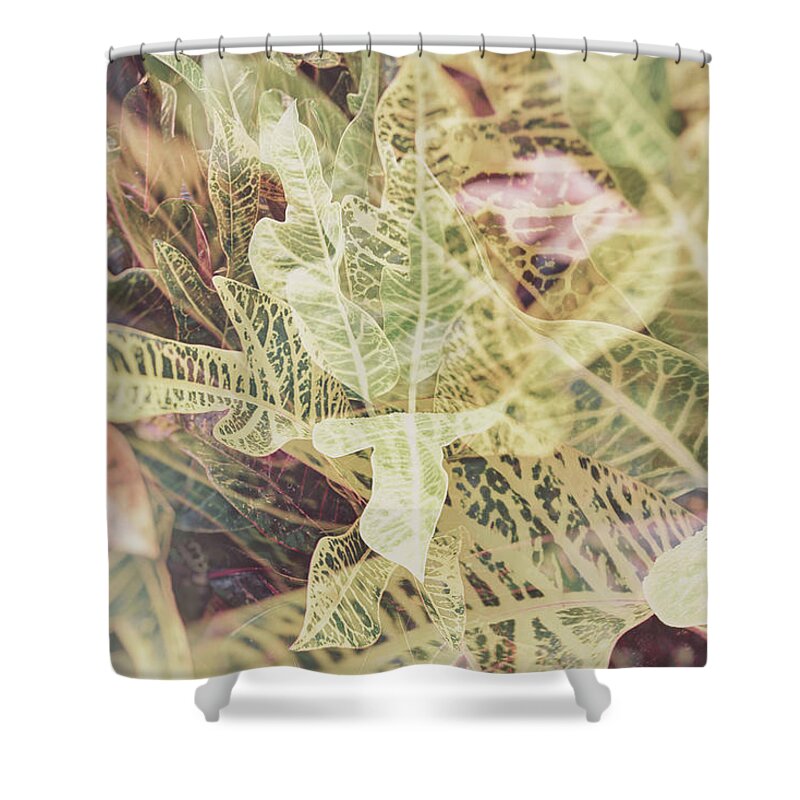This product photograph showcases a square-shaped shower curtain adorned with a detailed and artistic leaf pattern. The curtain, fully stretched taut across a slightly curved metal shower rod, is attached with around ten silver rings. The top of the image prominently features the curved rod, while the bottom reveals the iconic white claw feet of a bathtub, largely hidden behind the curtain itself. 

The shower curtain's design is a sophisticated blend of muted, faded green, and grayish-green hues, depicting variegated, forked T-shaped leaves that appear to radiate outward from the center. The central perspective of the design mimics the view from above a plant, giving a sense of natural growth. 

Scattered across the curtain, the leaf imagery varies in focus and intensity, suggesting a dynamic, multimedia art approach. Some leaves are in sharp focus, while others are softer, contributing to a layered, almost chaotic composition. Predominantly green, the leaves also exhibit subtle yellowish tones, with occasional hints of purple, pink, and white, enhancing the overall artistic complexity of the design.